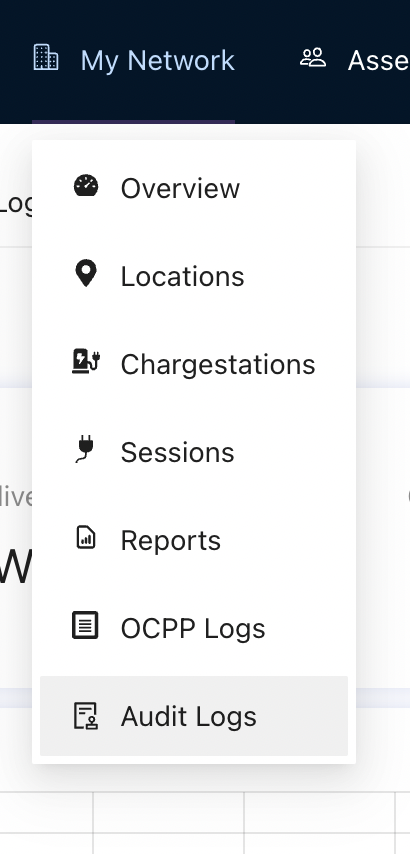The image depicts a pop-up window within an application interface titled "My Network." At the top-left corner, there is a small icon of two buildings, symbolizing networking or infrastructure. The pop-up menu presents a series of selectable options: "Overview," "Locations," "Charge Stations," "Sessions," "Reports," "OCPP Logs," and "Audit Logs." The "Audit Logs" option is distinguished by a light gray highlight, indicating it is the currently selected option. Each menu item represents a different function or data set available for user interaction within the app, providing a comprehensive suite of network management tools.